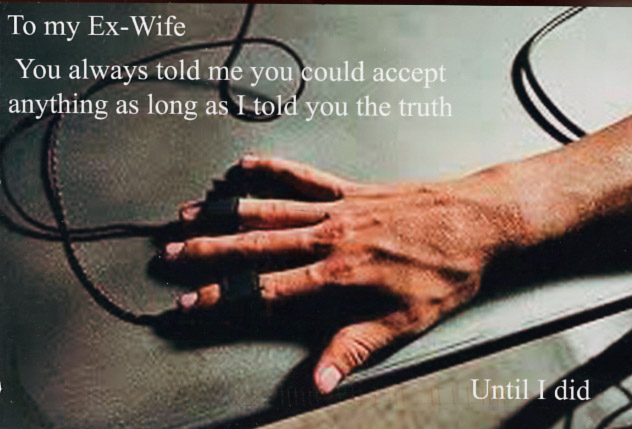A grainy, amateur-produced meme features the close-up of a lighter-skinned person’s hand, prominently displaying their veins. The hand rests on a black table, and around several fingers are attachments from lie detector equipment, with black sensors and visible wires casting shadows on the table. The background reveals a portion of the floor, and light reflects off the table’s surface. The image carries a poignant message in white font: at the top, "To my ex-wife, you always told me you could accept anything as long as I told you the truth," and at the bottom, "Until I did." The focus remains solely on the hand and part of the forearm, with no other visible text or objects.